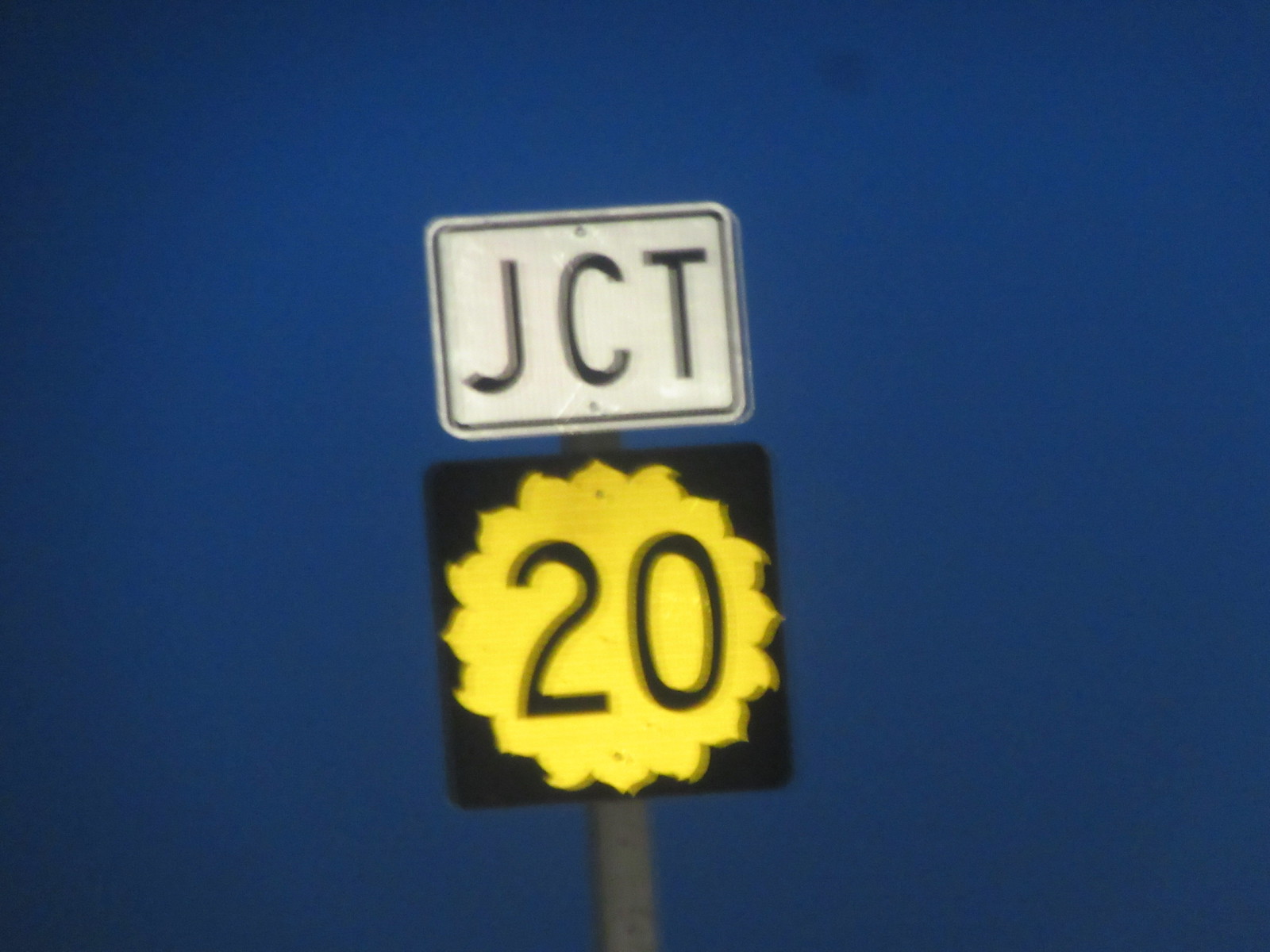This image captures a pair of road signs mounted on a single pole that extends nearly to the top of the frame. The upper sign is rectangular, featuring the letters "JCT" in bold, uppercase black text on a white background, bordered by a black band. Below it, the second sign is square-shaped with a black background, adorned by a spiky circular emblem resembling a stylized sun, at the center of which the number "20" is prominently displayed. The backdrop of the scene reveals a deep, dark blue sky, suggesting either twilight or early night, against which the well-lit signs stand out crisply.